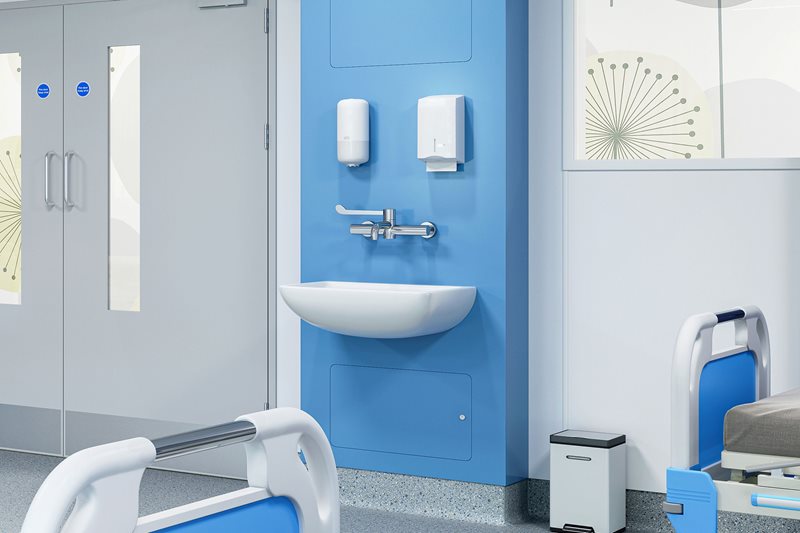The image depicts a meticulously detailed hospital room interior. On the left side, there are two gray double doors, each featuring a narrow, rectangular window covered to prevent visibility. Adjacent to the doors is a bright blue wall adorned with a white porcelain sink, mounted with a chrome-colored silver faucet. Above the sink, a soap dispenser and a paper towel dispenser are fixed to the wall. To the right of this sink, another covered window allows light in but obstructs the view. Below this window, there is a trash can positioned near the end of a hospital bed. This bed showcases a blue insert encased in white metal with a visible mattress. A similar hospital bed is situated on the left side of the room. The floor is a speckled gray, resembling poured tile. The remaining walls are painted a very light gray, contrasting with the medium blue feature wall. The room captures the sterile and organized environment typical of a medical institution.